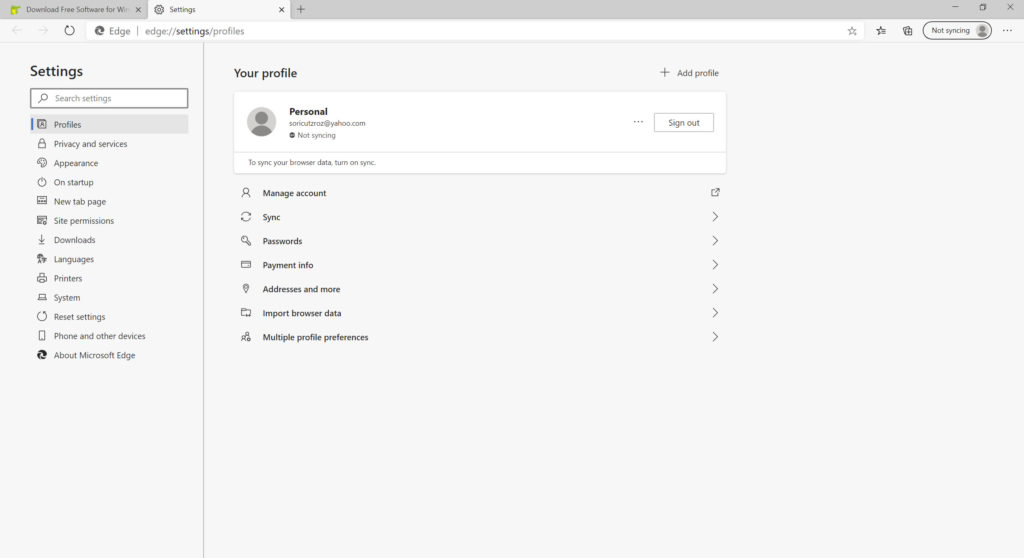This image captures a screenshot of the Edge browser, evident from the word "Edge" visible in the address bar, which reads "edge://settings/profiles." The top bar is gray, featuring the browser window controls (X, maximize, and minimize) on the upper right-hand side. Two tabs are open.

The main content of the browser displays the vertical settings menu on the left side, with the "Profiles" section open. To the right, detailed user profile settings are visible, labeled as "Personal." Below the profile label, options such as "Manage account" are present. Further down, there are several settings categories with corresponding arrows indicating expandable options, including "Sync," "Passwords," "Payment info," "Addresses and more," "Import browser data," and "Multiple profile preferences."